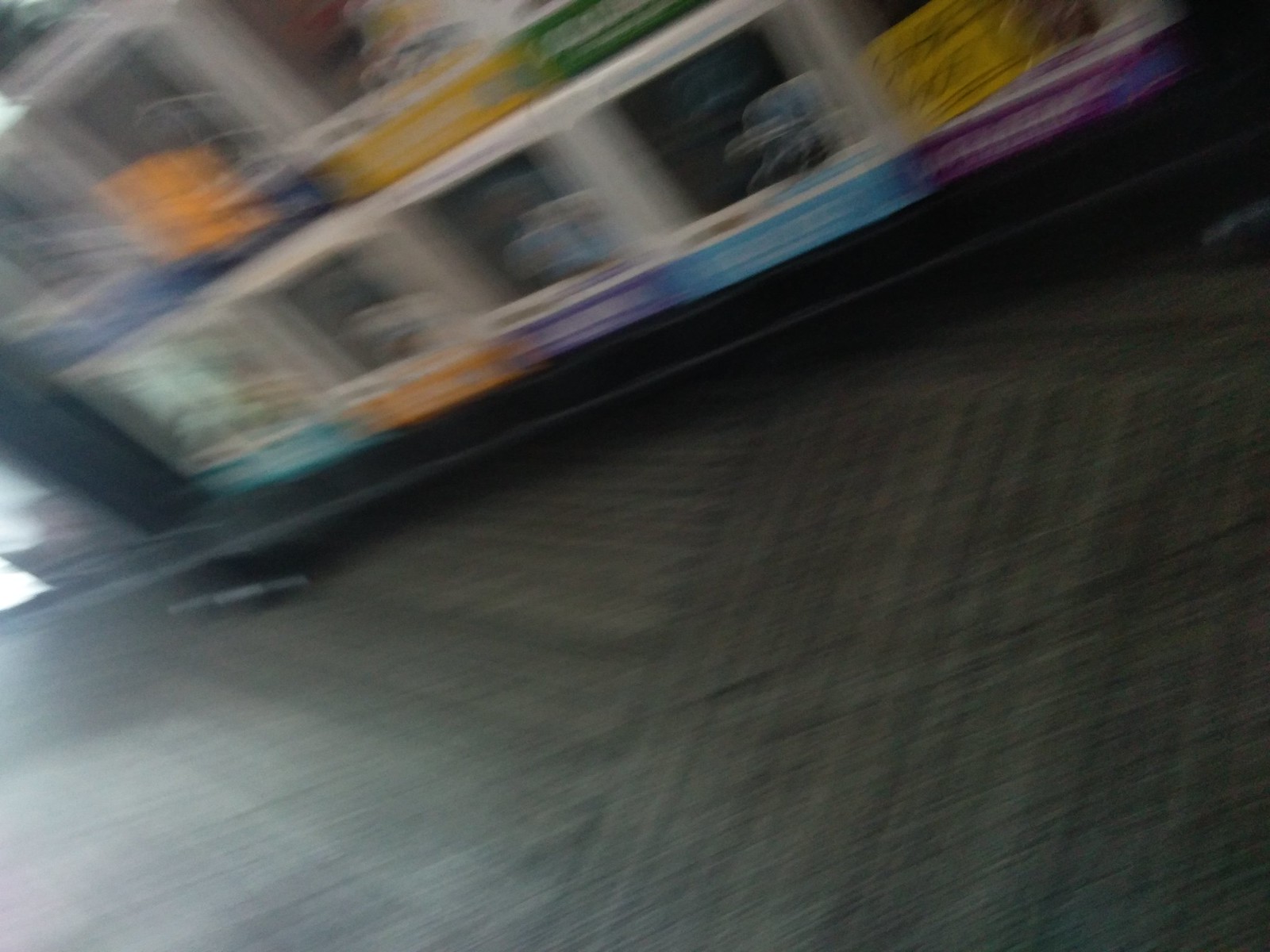The image is quite blurry, and it appears to have been taken while in motion, making it challenging to discern specific details. The focal point seems to be a cabinet with various enclosures, each designed to hold different items. Some of the enclosures contain objects that resemble Legos or other small, assorted items. There are promotional stickers affixed to some of the enclosures, suggesting the cabinet is intended for customer use, likely allowing individuals to select items directly. The enclosures are highlighted with colors beneath them to attract attention and enhance visual appeal. However, due to the poor image quality, the exact contents of the enclosures remain unclear.